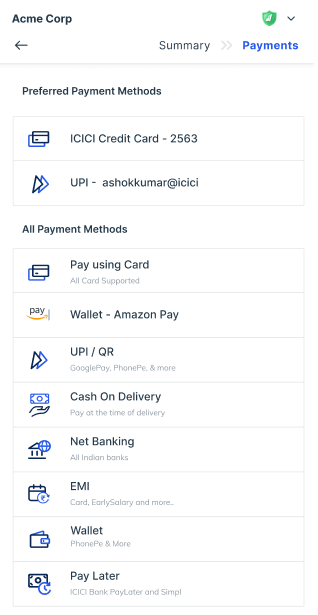Screenshot of a web page or app with an all-white background, titled "Acme Corp" in the top left corner. On the right-hand side, there's a green badge with a white icon inside and a drop-down arrow. Below this, on the left side, there's a left-pointing arrow. To the right, headings "Summary" and "Payments" are displayed, with "Payments" highlighted in blue, indicating it's currently selected.

The section beneath is labeled "Preferred Payment Methods," displaying an icon for a credit card followed by the text "ICICI Credit Card 2563." Below this, another method is listed with two triangles icon and the text "UPI ashokkumar@icici."

Further down is the heading "All Payment Methods," listing a variety of options:
1. **Credit Cards**: A selection to "Pay Using Card - All Cards Supported."
2. **Amazon Pay**: An option with the Amazon logo, labeled "Wallet - Amazon Pay."
3. **UPI**: Displayed with two triangles, followed by "UPI shokumar, Google Pay, PhonePe, and more."
4. **Cash on Delivery**: Indicated with a dollar bill and a hand icon, labeled "Pay at the Time of Delivery."
5. **Net Banking**: Represented with a bank icon and the text "All Indian Banks."
6. **EMI**: Displayed with a card icon and labeled "Card, Early Salary, and more."
7. **Wallet**: Shown with a wallet icon and the text "PhonePe, Mobikwik, and more."
8. **Pay Later**: Indicated with a dollar icon and the text "Post-Purchase Payment Options."

These options provide users with a diverse and detailed choice for completing their payment transactions.